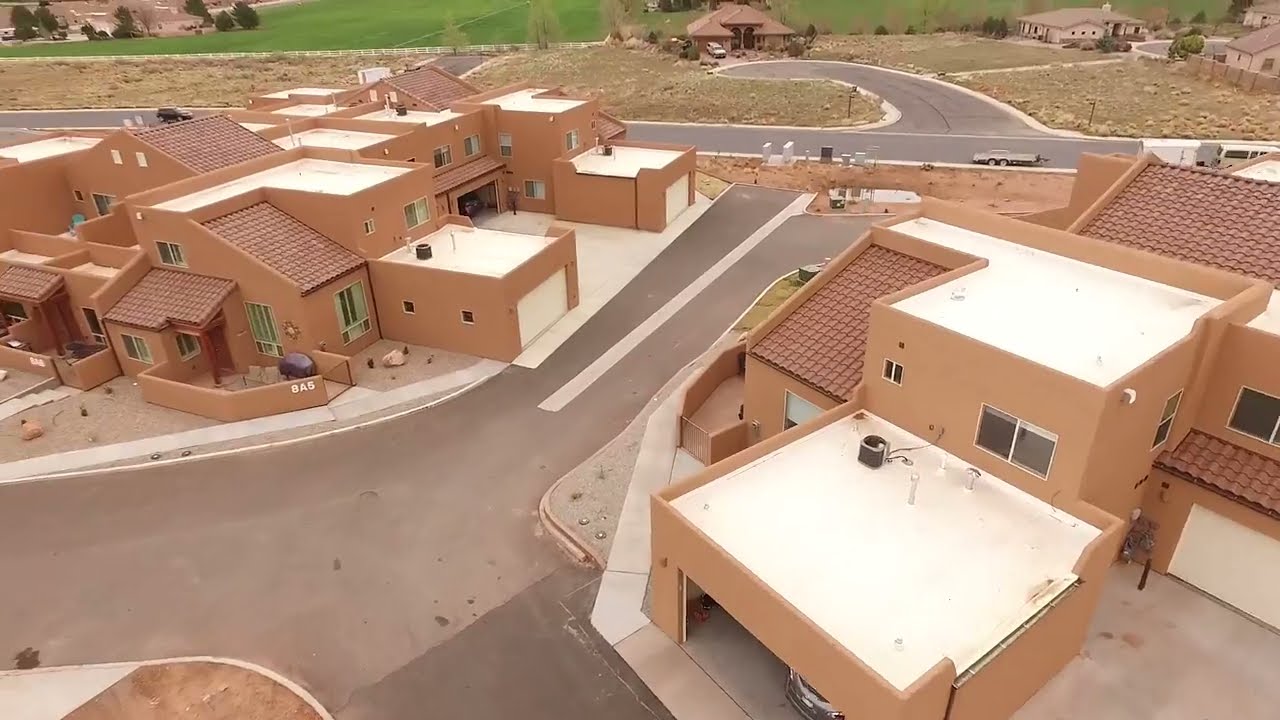In this daytime bird’s-eye view, a smiling woman stands on red clay sand, looking directly up at a drone capturing her selfie. She has black hair tied back in a ponytail and is wearing a black sweatshirt with gray stripes along the sleeves and shoulders. She sports brown-lensed sunglasses and holds what appears to be a controller or smartphone in her left hand. At her feet, there is a small white radio-controlled truck, while another blue remote-control truck can be seen in the upper left corner of the image. To her left, a large tumbleweed is prominent, with additional smaller tumbleweeds and brambles scattered around. The scene suggests an arid environment, possibly a desert.